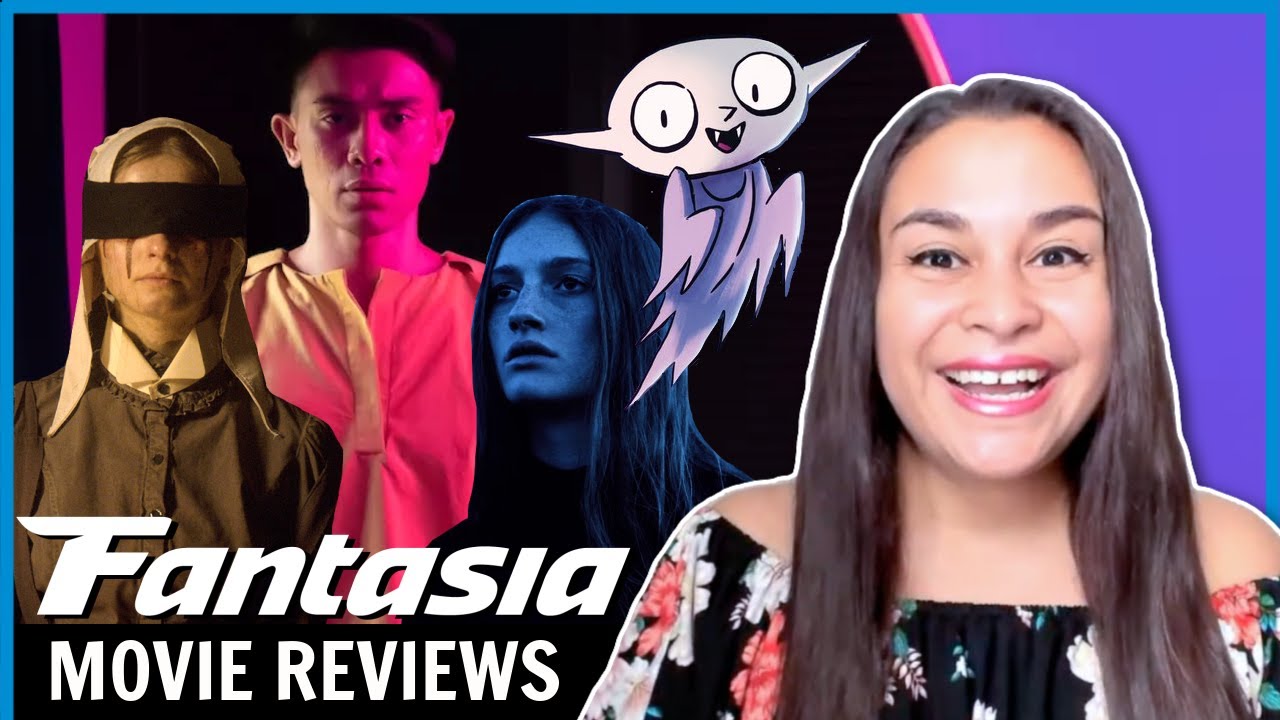This image appears to be a promotional thumbnail, potentially from a YouTube channel or a similar website, titled "Fantasia Movie Reviews," as indicated by the white font in the bottom-left corner. The focal point is a smiling young woman, likely of Hispanic descent, with long brown hair. She is dressed in an off-the-shoulder floral top, which is mostly black with colorful flowers. Positioned against a backdrop featuring various movie characters, the image has a homemade, flyer-like quality.

The woman, presumably named Fantasia, appears joyful and exudes a vibrant persona. To her right, a series of movie characters serve as a testament to her reviews. The characters depicted include: a bonnet-wearing female figure with a light-colored bonnet and blacked-out eyes; a male character with dark hair, possibly of Asian descent, dressed in a white top; a white woman with dark hair viewed through a black-and-white filter, facing left; and finally, a simply drawn cartoon character reminiscent of Nosferatu, smiling in a sidekick-like manner. Each character is set against distinct color themes, enhancing the collage's visual appeal and suggesting diversity in the films reviewed by Fantasia.